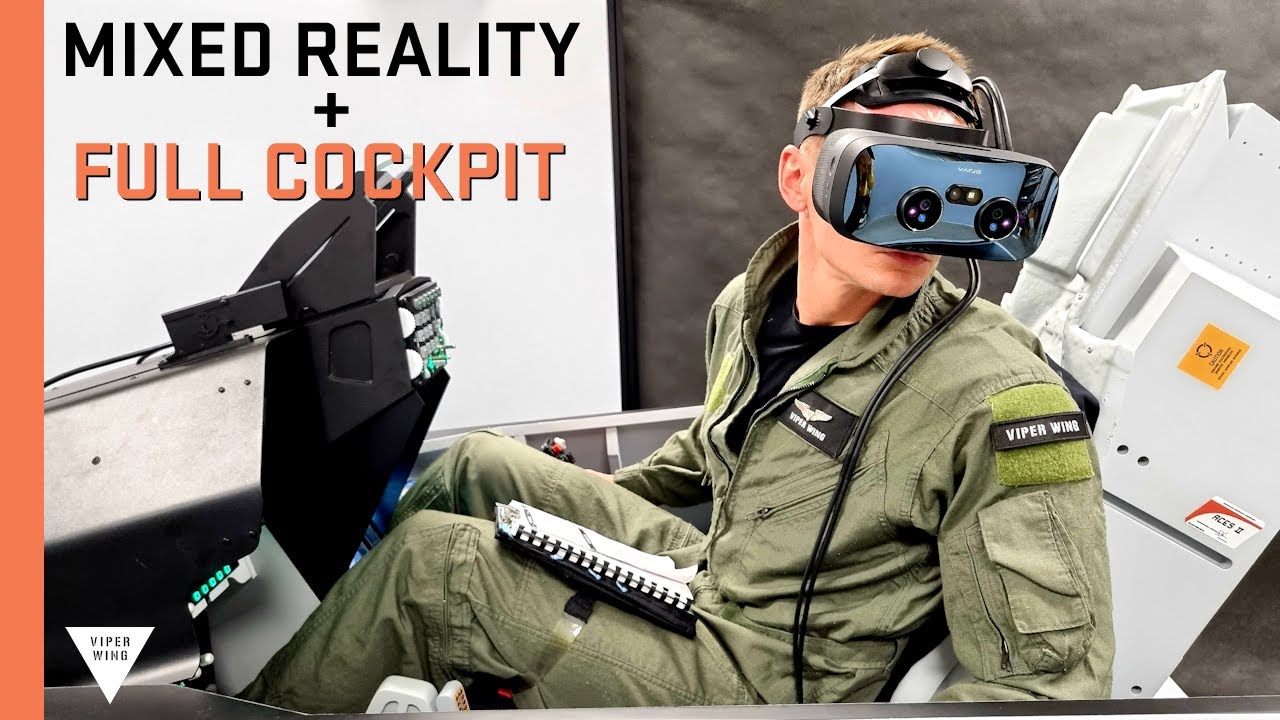This image is a detailed advertisement featuring a young man in a mixed reality training setup. The man is seated in a mock-up cockpit, wearing an olive green flight suit with logos, including one that reads "Viper Wing" and golden wings on his chest, suggesting a military or aviation context. His suit has a one-piece, zip-up design typical of pilot uniforms, and there is a white pad with black rings on his lap, likely for instructions.

He is equipped with a virtual reality headset, complete with black wires trailing over his left shoulder. The VR setup is designed to simulate a full cockpit experience, as indicated by the text on the left side of the image, which reads "MIXED REALITY + FULL COCKPIT" in black and orange. He's seated in a white chair with a black control console in front of him, designed to mimic plane controls. The advertisement is set against a gray background, with an orange stripe running down the left side, giving it a modern, high-tech appearance.

In the bottom left corner, an upside-down triangle logo for "Viper Wing" is displayed, reinforcing the branding and purpose of this training device. The man's intent posture and the immersive setup emphasize the advanced, realistic nature of the training simulation.